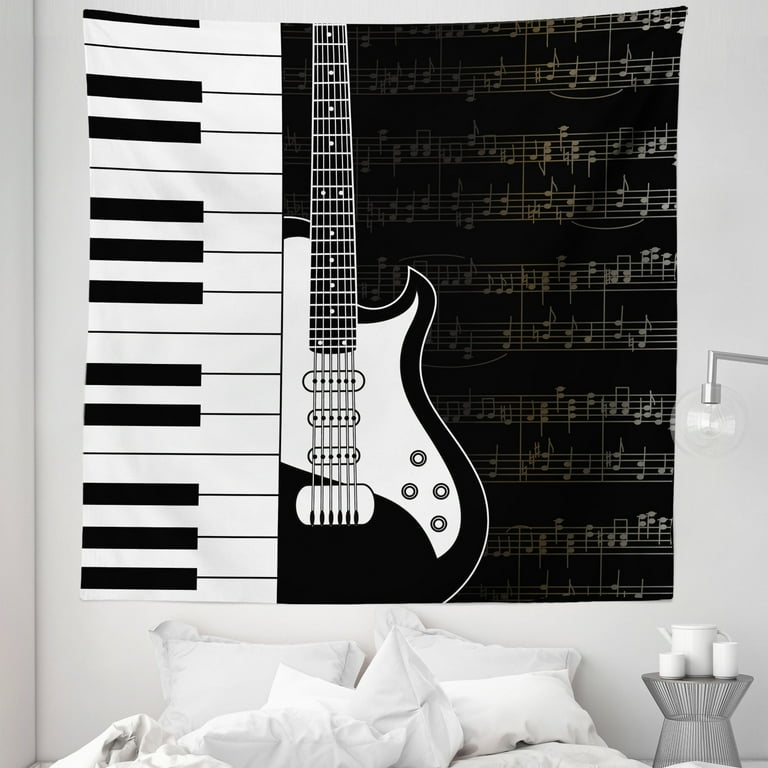This color photograph captures a serene bedroom with predominantly black and white elements. The focal point is a bed with ruffled white sheets and four pristine white pillows. Beside the bed stands a uniquely shaped nightstand, described as a combination of trapezoidal structures, supporting two white cups and a small white pitcher. A sleek, silver desk lamp with a clear bulb is positioned on the right side of the nightstand. Dominating the white wall above the bed is a large, striking poster featuring vertical piano keys on the left, a centrally placed white and black guitar, and musical notes on a black background to the right. The overall aesthetic of the room is clean and musically themed, creating a monochromatic yet harmonious ambiance.